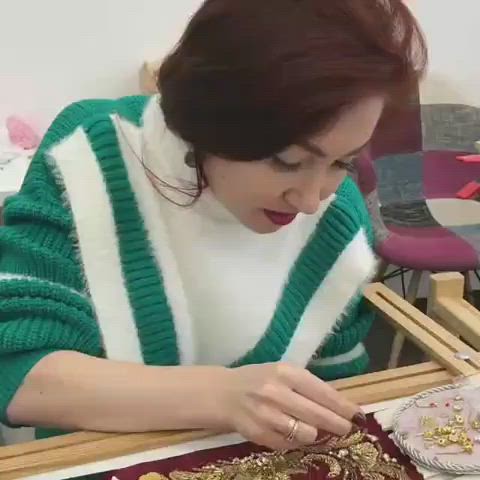The photograph features a young woman with medium-length auburn hair, styled in a way that highlights its reddish hue. She is slightly facing to the right, leaning over a wooden table as she closely inspects a piece of red fabric adorned with gold embroidery, possibly engaged in some intricate beadwork or decorative craft. Her right hand, which is in focus, reveals maroon-painted nails and a ring, delicately touching the material. She is dressed in a cozy green and white sweater over a white shirt. The background showcases a light-colored wall over her right shoulder and a multicolored chair with wooden legs to her right. The table she is working on appears to have a unique design, featuring two intersecting wooden bars connected by a metal rivet, suggesting it's specialized for craftwork. Additional white material extends off the right side of the image, adding to the scene’s detail.